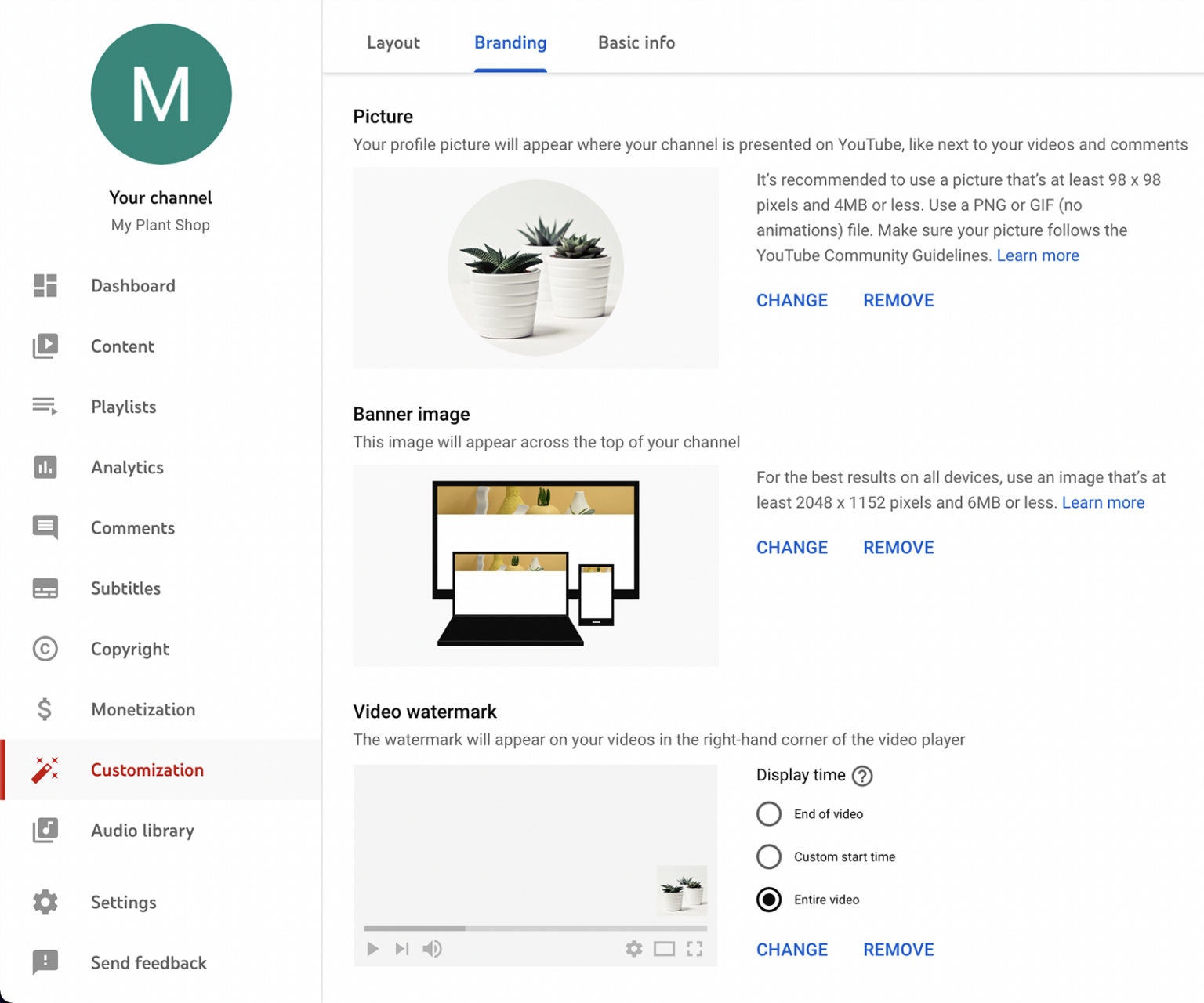This detailed caption describes a webpage interface, specifically a content management system for a plant shop's YouTube channel layout customization:

---

On the left-hand side of the webpage, there is a prominent green circle containing a bold white "M." Directly beneath this, bold black text reads "Your Channel," followed by grey text stating "My Plant Shop." The left-hand menu contains various icons and their corresponding labels:

1. **Dashboard**: Represented by a square icon constructed from two rectangles and two smaller squares with narrow spacing.
2. **Content**: Depicted by an icon of two overlapping squares, one featuring a white triangle.
3. **Playlist**: Illustrated with three horizontal lines and an arrow.
4. **Analytics**: Shown as a black square with a white bar graph.
5. **Comments**: Represented by a chat bubble with white lines.
6. **Subtitles**: Displayed as a square containing smaller white squares.
7. **Copyright**: Illustrated by a circle with a "C" inside.
8. **Monetization**: Indicated by a money symbol.
9. **Customization**: Highlighted with a magic wand icon featuring three stars. This section is currently selected, evident by its red outline and light grey background, with the black text turning red.
10. **Audio Library**: Depicted as two squares, the upper one containing a music symbol with a dark grey background.
11. **Settings**: Represented by a gear icon.
12. **Send Feedback**: Illustrated by a thought bubble with an exclamation mark.

On the right-hand side of the white content area, the interface reads "Layout" in black, followed by "Branding" in blue with an underline, signifying it is the active selection. "Basic Info" appears in black below.

Within the "Picture" section, there are images showing white potted plants with green foliage. Under "Banner Image," there are mockups of the webpage on a laptop, desktop, and smartphone. 

The "Video Framework" section features a rectangular thumbnail with the same white pots and green plants. This resembles a YouTube video interface, complete with playback controls: a play button, jump forward button, audio control, a gear icon, a small square for window expansion, and a larger square with L-brackets for fullscreen mode.

On the right side, options listed include "Display Time" in bold white and black text, accompanied by a grey question mark. Three selectable circles provide further options: "End of Video," "Custom Start Time," and "Entire Video," which is currently selected. Each option includes hyperlinked text in blue bold for "Change" and "Remove," with the first two options also stating "Learn More" in hypertext blue at the end of their respective paragraphs.

---